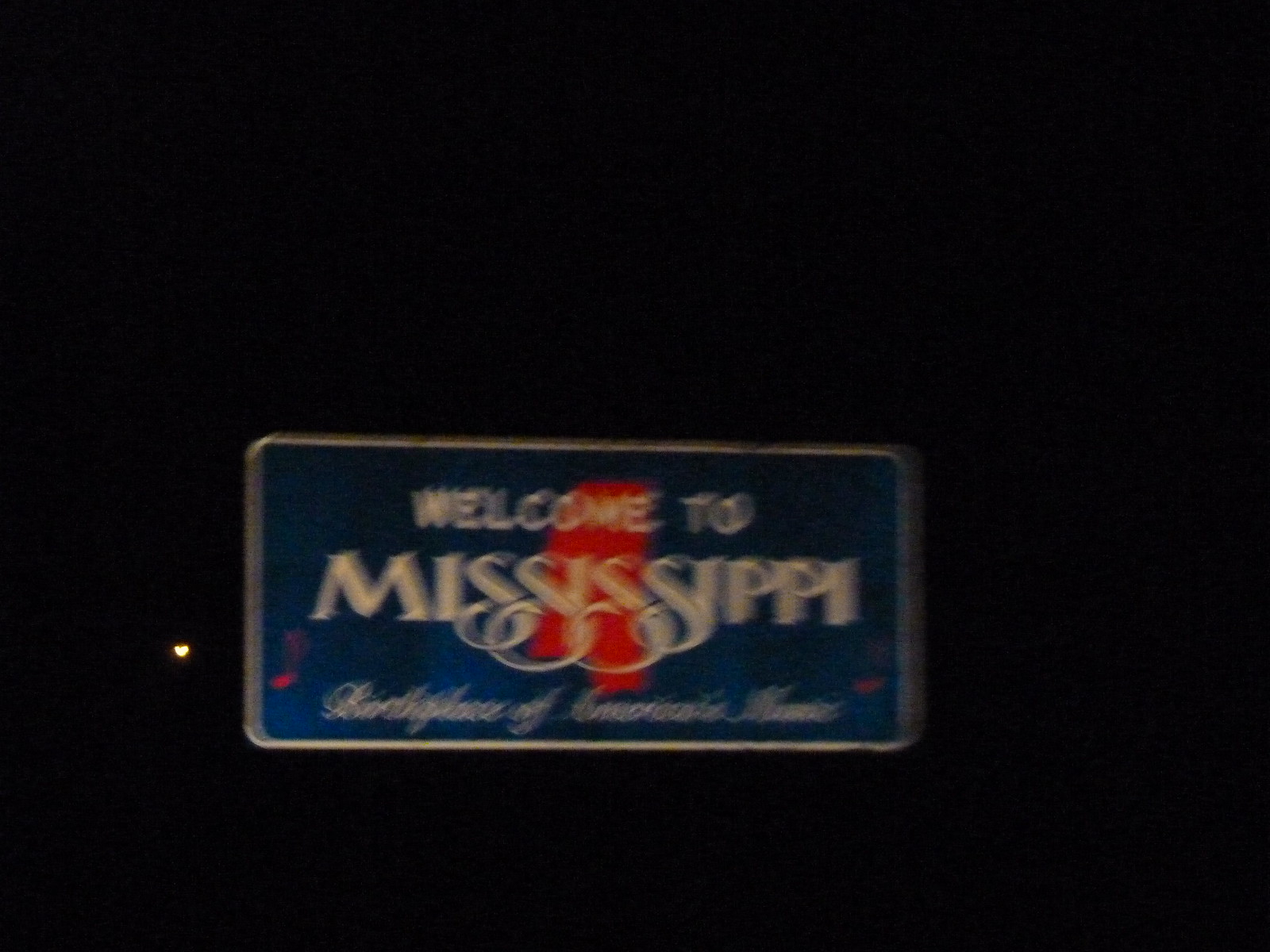A slightly grainy nighttime photograph captures a prominent blue sign with a thin white border that appears somewhat dirty. The sign reads "Welcome to Mississippi" in bold white font. Below this, there is a hard-to-decipher cursive script, also in white. Positioned on the sign is an outline of the state of Mississippi highlighted in red. Adding a touch of musical charm, red music notes adorn both sides of the sign. Off to one side of the image, a light casts a whitish-amber glow, adding to the nighttime ambiance. The overall image is somewhat blurry, with no other objects present.